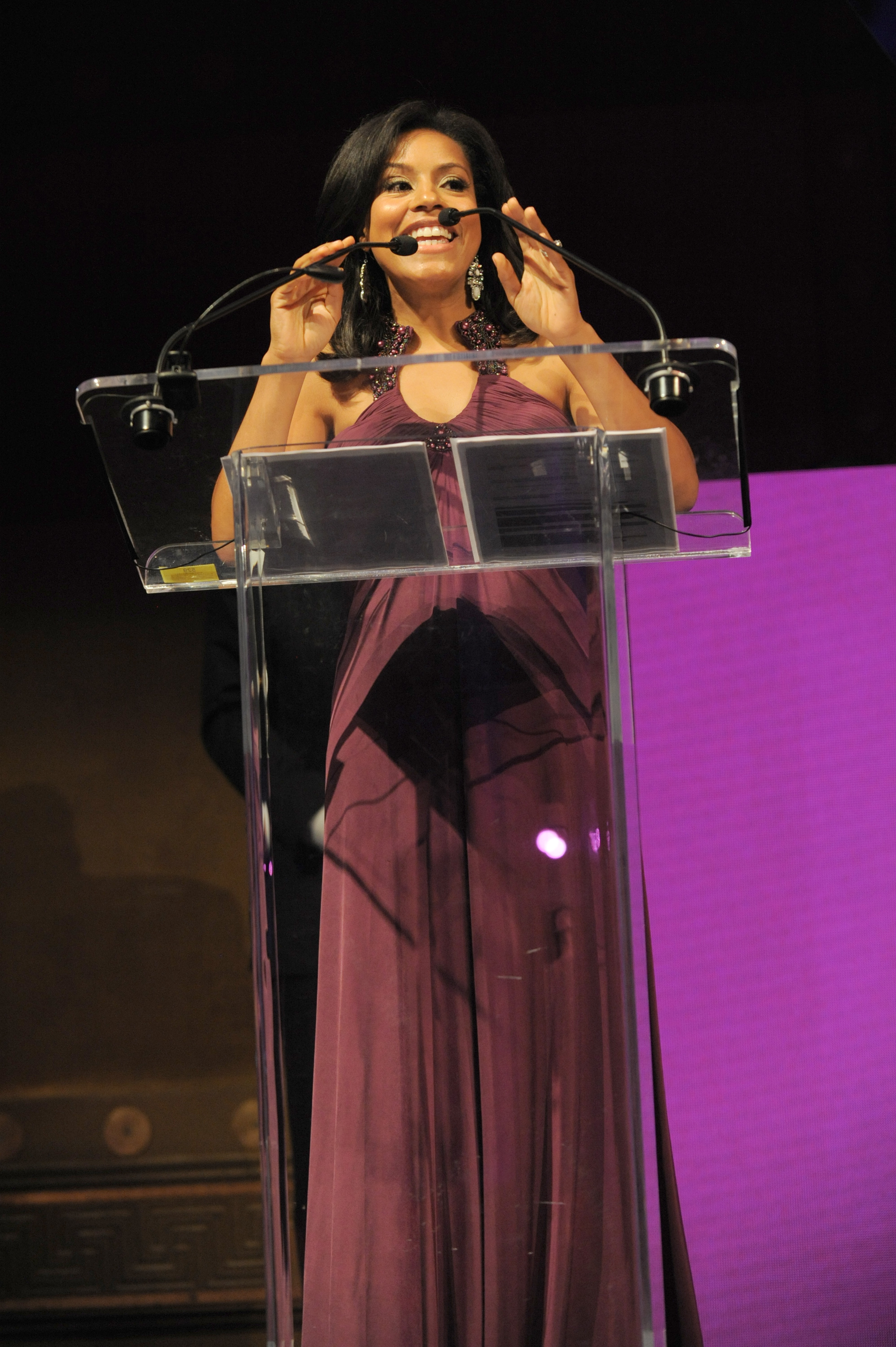This horizontally aligned photograph captures a poised woman at what appears to be an awards ceremony, either giving or accepting an award or making an announcement. She is positioned behind a tall, mostly clear podium, through which her maroon sleeveless evening gown is visible. The dress, made possibly from cotton, linen, or a blend, is detailed with several creases, including a prominent vertical line running from beneath her chest down the belly, flanked by perpendicular creases.

The woman is smiling, with a space between her upper and lower teeth visible, and is looking slightly upward to her right. She has smooth, shoulder-length black hair and a tan or mocha-colored complexion. Her hands are elegantly resting on the microphone stands, which are angled towards her face, holding up three microphones with small black bulbs on top. She also wears eye-catching, glamorous earrings, possibly diamond or rhinestone, approximately the size of two quarters each.

The background on the right side of the image features a bright magenta screen while the upper part merges into shadows. To the left, there's a complex pattern with rectangular, up-down, up-down shapes and small metallic-looking decorative elements. There are also two pieces of paper on the podium, and a yellow object, perhaps a pen or highlighter.

Despite the shadows and light peach and gray hues in parts of the background, the overall scene is clearly visible, capturing the woman's elegant demeanor and the possible excitement of the moment. This prominent figure, recognizable to some as a morning host from Good Morning America, exemplifies grace and confidence during what seems to be a notable event.